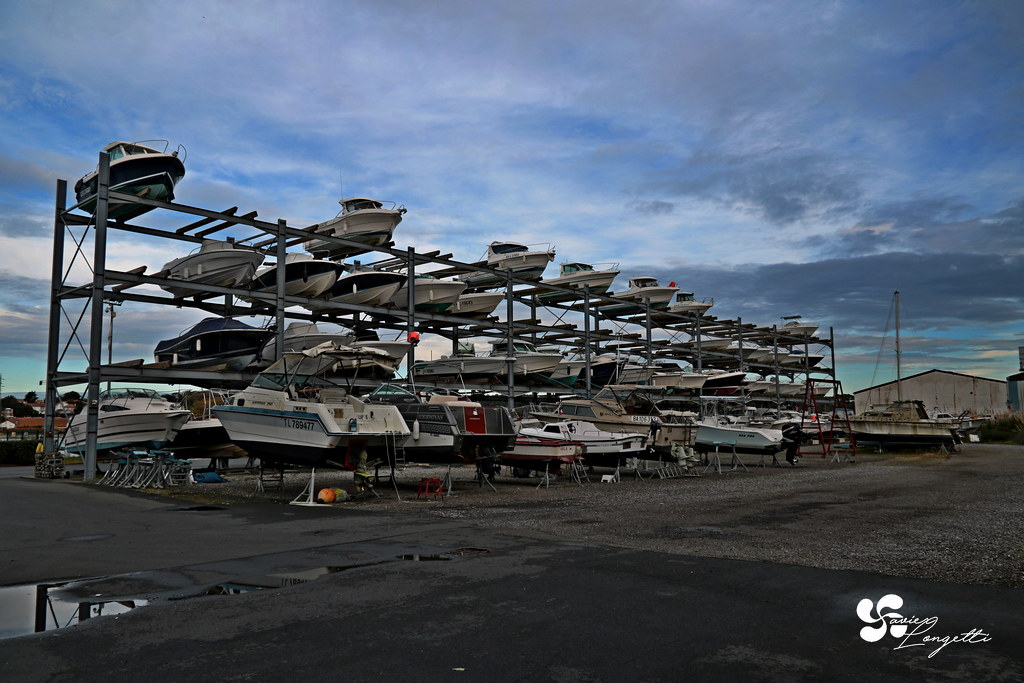The image depicts a boat storage yard on a partly cloudy day, with signs of recent rainfall indicated by puddles on the blacktar pavement. The focal point is a large metal rack situated near the center, holding approximately 40-50 smaller boats, primarily fishing and pleasure boats. These boats are neatly arranged for long-term storage, while a few larger boats are positioned on stilts nearby. To the right, a gray warehouse stands prominently, contrasting with the newer, darker pavement on the left side of the image. In the bottom right corner, there is a logo in white cursive writing, though its text is difficult to decipher. The sky transitions from a clear blue with thin white clouds at the top to darker gray clouds near the horizon, suggesting incoming or recently departed rain. Additionally, hints of a fishing community can be glimpsed in the distance to the left, enhancing the scene’s maritime atmosphere.